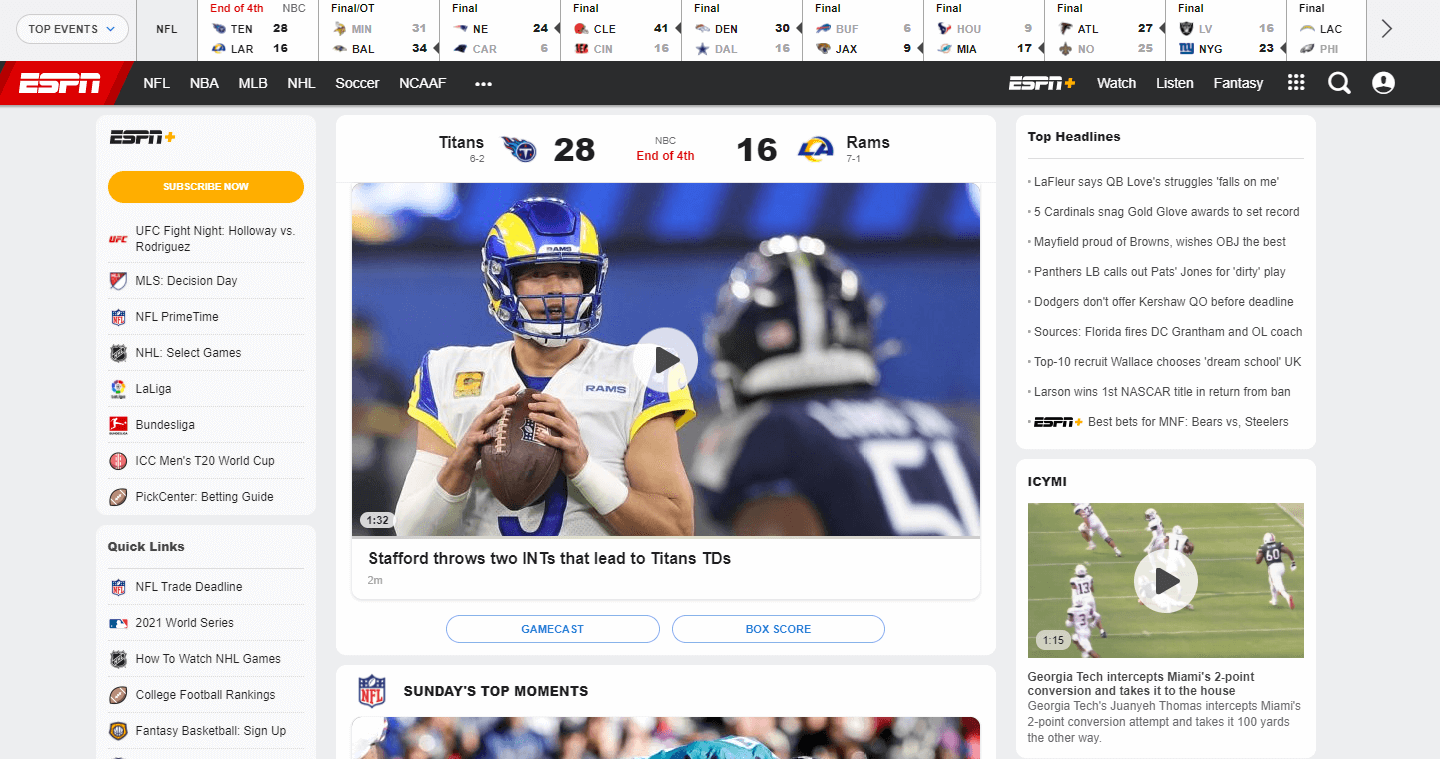The image is a screenshot of the ESPN website. In the top left-hand corner, there's a white oval labeled "Top Events" with a dropdown arrow next to it. To its right, the heading "NFL" is prominently displayed. Below this, there's a scoreboard section featuring various team icons and scores. The Tennessee Titans' icon is distinguishable, followed by the abbreviation "LAR", indicating the Los Angeles Rams. The "End of the 4th" quarter status is marked in red, suggesting a recently concluded game. On the right side, the word "Final" indicates completed matches, showing a score of 34 between Minnesota and Baltimore, highlighted in black. The layout continues in this format, listing other teams, such as the Los Angeles Chargers (LAC) and Philadelphia Eagles (PHI), identified by their respective icons.

To the right of this scoreboard section, there's an arrow allowing users to navigate the carousel of scores. Below this main section, within a black banner on the left side, the ESPN logo is situated, followed by menu options like NFL, NBA, MLB, NHL, soccer, and NCAAF, with three dots on the right for additional options. This menu also includes links labeled ESPN+, Watch, Listen, Fantasy, and various icons for related content.

Underneath the navigation menu, a media image features football gameplay, depicting a quarterback and an approaching defender, with a caption reading "Titans 28, Rams 16." To the right, the Top Headlines section appears, containing another media image of a video. On the far left, there's a "Subscribe Now" prompt accompanied by icons related to different categories.